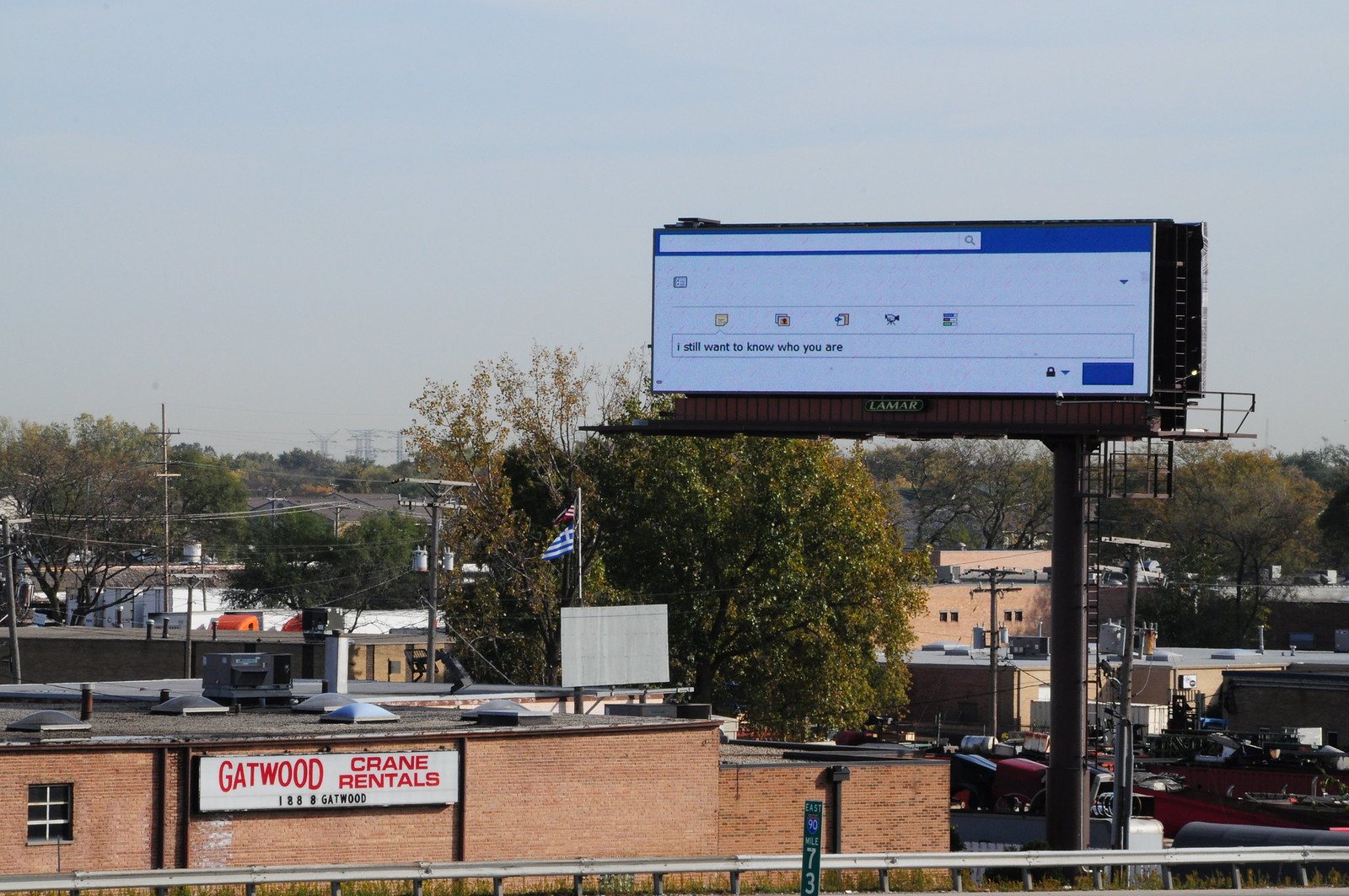In this photograph of an urban area viewed from an elevated roadway, we see a collection of several brown brick buildings typical of a manufacturing zone. Prominently, there is a building with a sign that reads "Gatwood Crane Rentals, 1888 Gatwood" in red lettering. Adjacent to this building rises a tall digital billboard, resembling a computer screen, and displaying the text "I still want to know who you are" in black. This billboard, a Lamar Brand, towers over nearby trees and electric poles with power lines. An American flag, accompanied by a second flag that appears to be Swedish, flutters on a flagpole behind the buildings. Various vehicles and trucks are parked around the area, indicating the busy nature of the locale. A mile marker with the number 73 is visible along the roadway, possibly indicating Route 80 in this business district of the town.